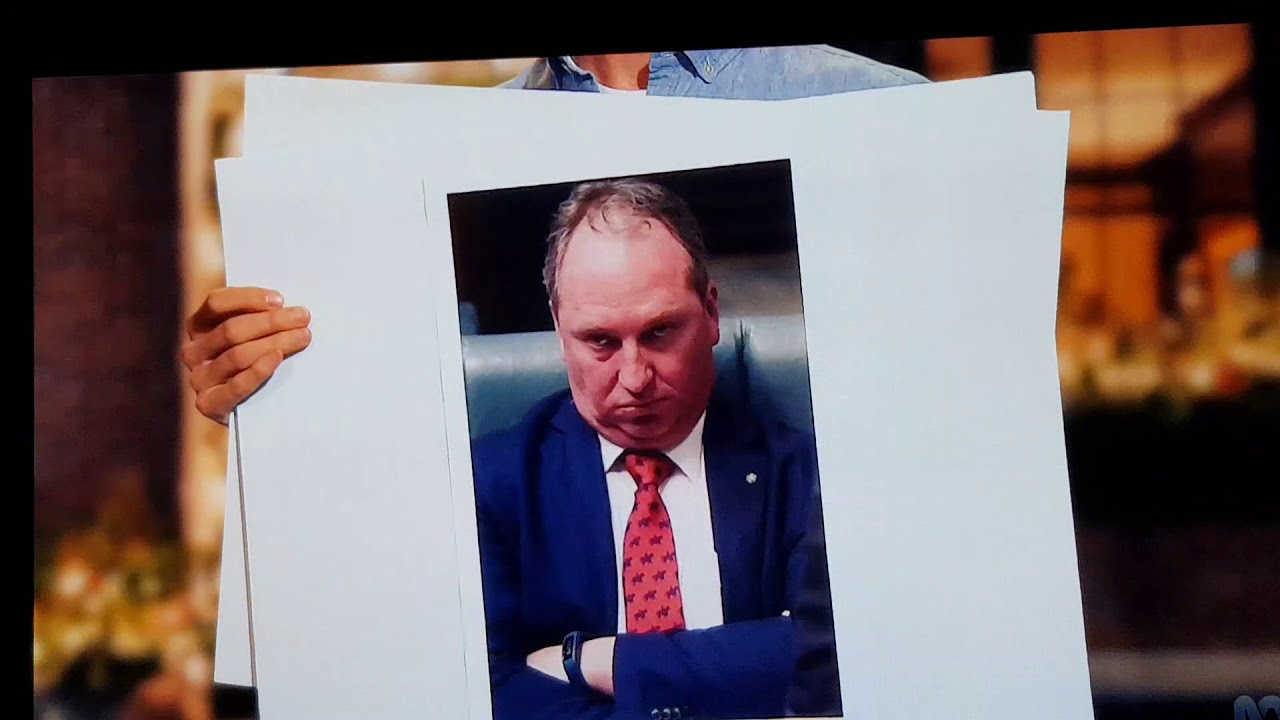The image depicts a person, whose face is not visible, holding two large white poster boards against a black background. The posters are slightly rotated counterclockwise. The person's right hand grips the left edge of the posters. Each poster bears a central photograph of a middle-aged, balding white man. This man, appearing slightly heavyset, is clad in a dark blue suit, a white dress shirt, and a pink tie with small, indistinct patterns that might be horses or stars. He sits in a plush blue chair with his arms crossed, exuding an air of frustration or worry as he looks down from underneath his eyebrows, accentuating his double chin. The overall scene bears a whimsical resemblance to the iconic moment from *Love Actually* where a character holds up message cards, but here, it is a grumpy businessman or politician featured prominently.